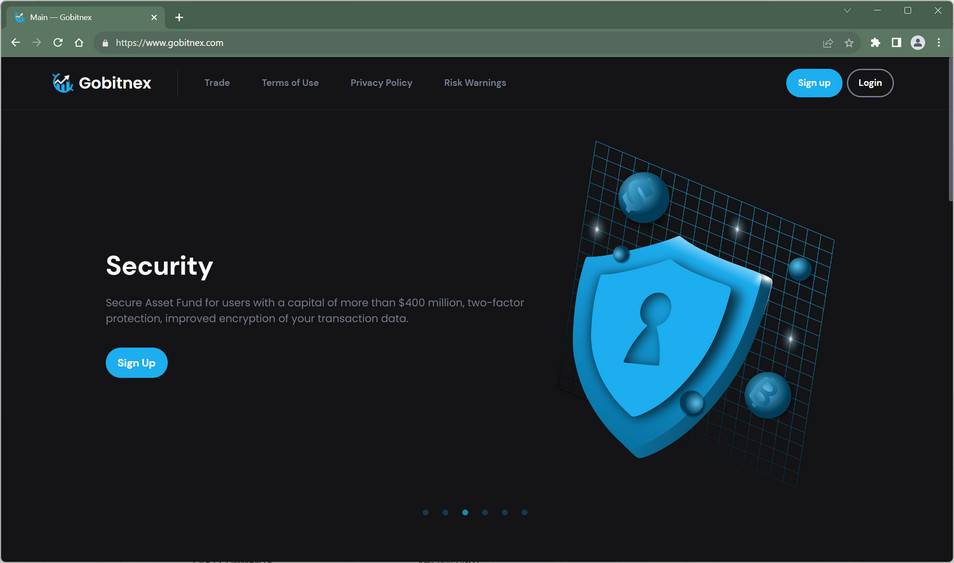The screenshot captures a webpage from the URL https://www.gobannex.com. At the top, the browser's header is colored greenish-gray with a tab displaying the title "Main Gob Annex." The center of the screen is dominated by a large black area. In the upper left corner, the text "Gob Annex" is prominently displayed in white. To the right of this header text are navigation links labeled "Trade," "Terms of Use," "Privacy Policy," and "Risk Warnings." On the far right side of the header are two action buttons: one blue button labeled "Sign Up" and a secondary button labeled "Log In."

On the left side of the screen, in a white font, is the heading "Security," which describes various security features offered by the site, including "Secure Asset Fund for Users with a Capital of more than $400 million," "Two-Factor Protection," and "Improved Encryption of your Transaction Data." Below this text is another blue "Sign Up" button.

The right side of the screen features a large image of a shield with a keyhole in the middle, symbolizing security. The background behind the shield consists of a grid of small squares, with two large, circular blue bubbles superimposed on it, each marked with the letter "B."